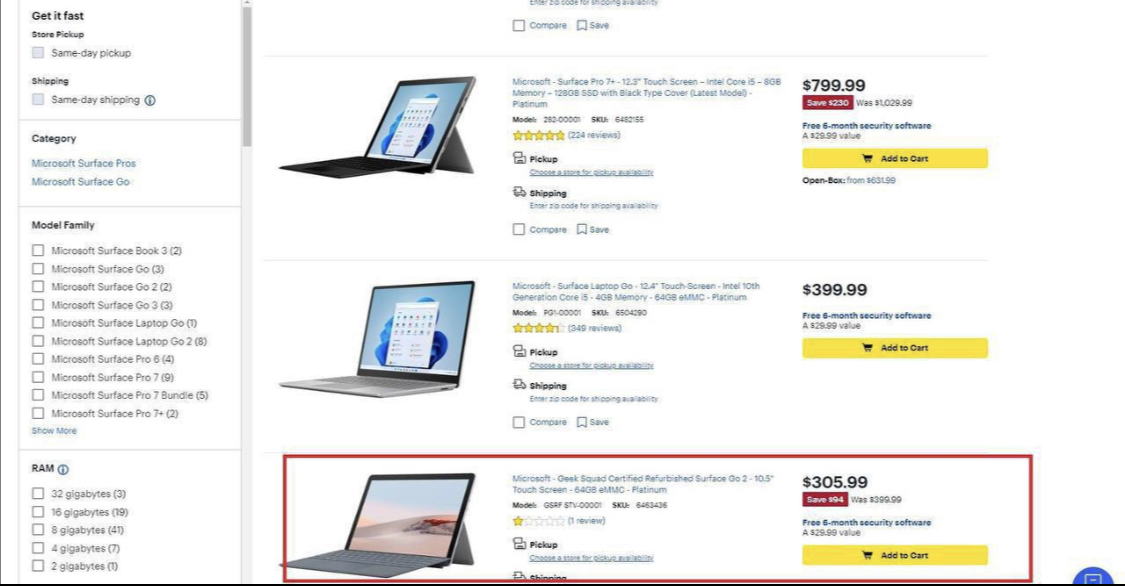The image is set against a white background, prominently featuring bold black text in the upper left corner that reads "Get it fast." Below this, there is a navigation menu with options labeled in black text as "Store Pickup," "Same-Day Pickup," "Shipping," and "Same-Day Shipping." Beneath the menu, the word "Category" appears in black text, followed by "Microsoft Surface Pros" and "Microsoft for Surface Go" in blue text. 

A gray horizontal line separates these elements from the next section, where "Model Family" is displayed in bold black text. Below this heading, a series of checkboxes list various models, including "Microsoft Surface Book 3," "Microsoft Surface Go," "Microsoft Surface Go 2," "Microsoft Surface Go 3," and "Microsoft Surface Laptop Go."

On the right side of the image, three color photographs of laptops are displayed. The bottom laptop is highlighted in red, indicating it has been chosen, and identified as "Microsoft Geek Squad Certified Refurbished Surface Go 2." The price for this model is shown as $305.99.